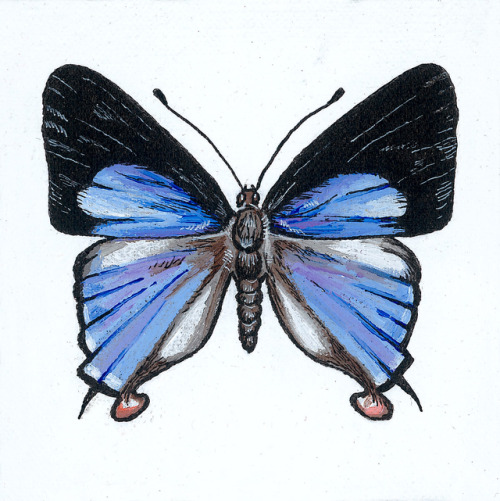The image is a detailed, brightly lit painting of a butterfly, viewed from a top-down perspective. The butterfly's body is primarily brown with some gray tinges, and it features long, black, moth-like antennas. The wings are vividly colored, showcasing a gradient from black at the edges to a spectrum of blue and purple towards the center. The upper wings have black edges with a small area of blue near the inner parts, while the lower wings display a blend of blue and purple hues. Additionally, there are touches of white and brown on the wings, with a slight brown tinge near the tips. The background is a clean white, accentuating the vibrant colors of the butterfly. The overall image is a watercolor illustration, and it captures the intricate details and natural beauty of the butterfly’s design.